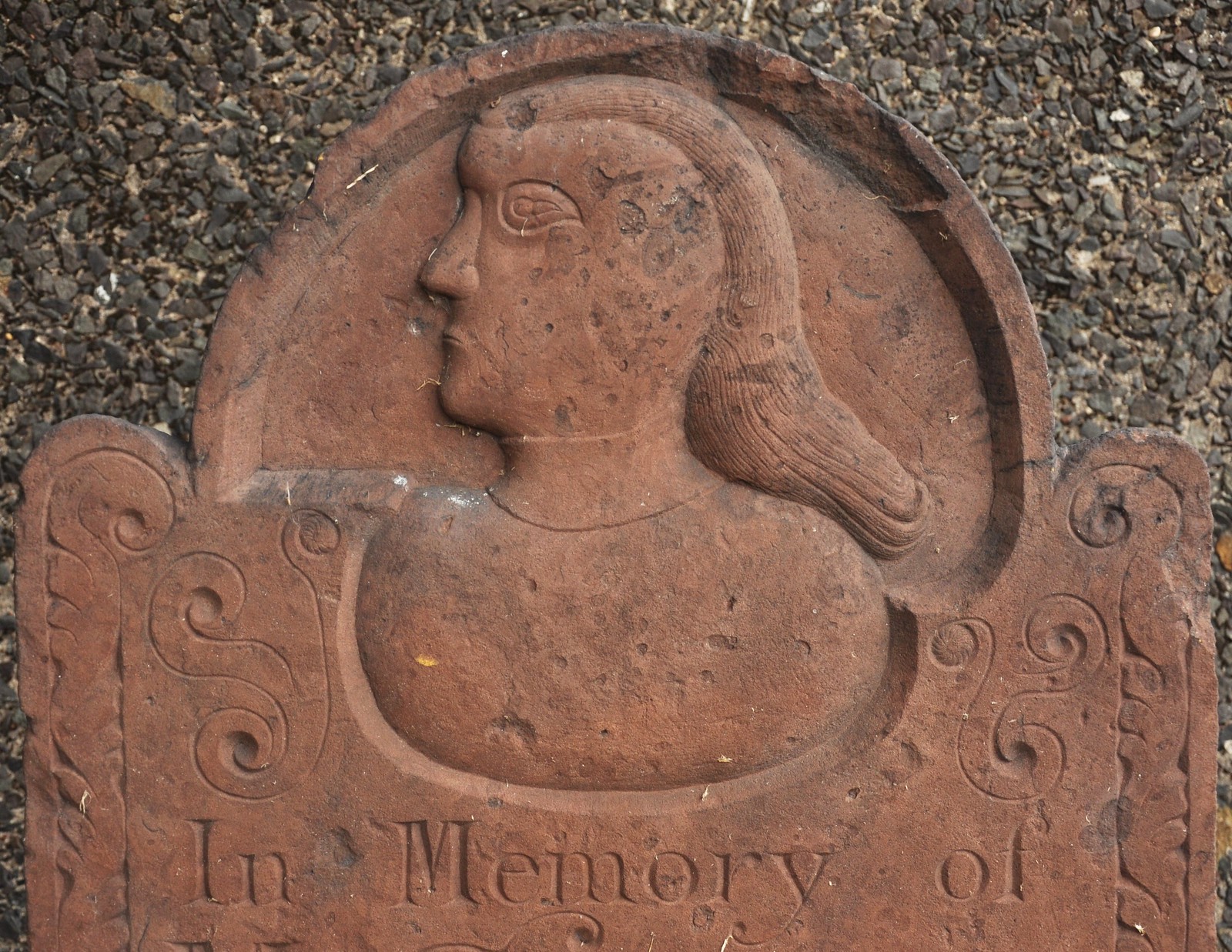The image depicts a weathered, horizontal, rectangular tombstone or memorial plaque made predominantly of brownish-red stone, eroded from the elements, indicating its age. The top of the tombstone features a carved profile of a woman or possibly a Roman-style gladiator looking to the left, with distinct features including a prominent nose, a large eye, long hair, and a small mouth. The figure appears to be wearing a large collar. The phrase "In Memory Of" is etched into the stone below the figure, although no further text is legible. The stone's surface is adorned with squiggly lines and patterns, adding to its intricate design. The tombstone is set against a backdrop of gray sediment and small pieces of gravel, suggesting a grave setting, with trees and leaves visible in the background.